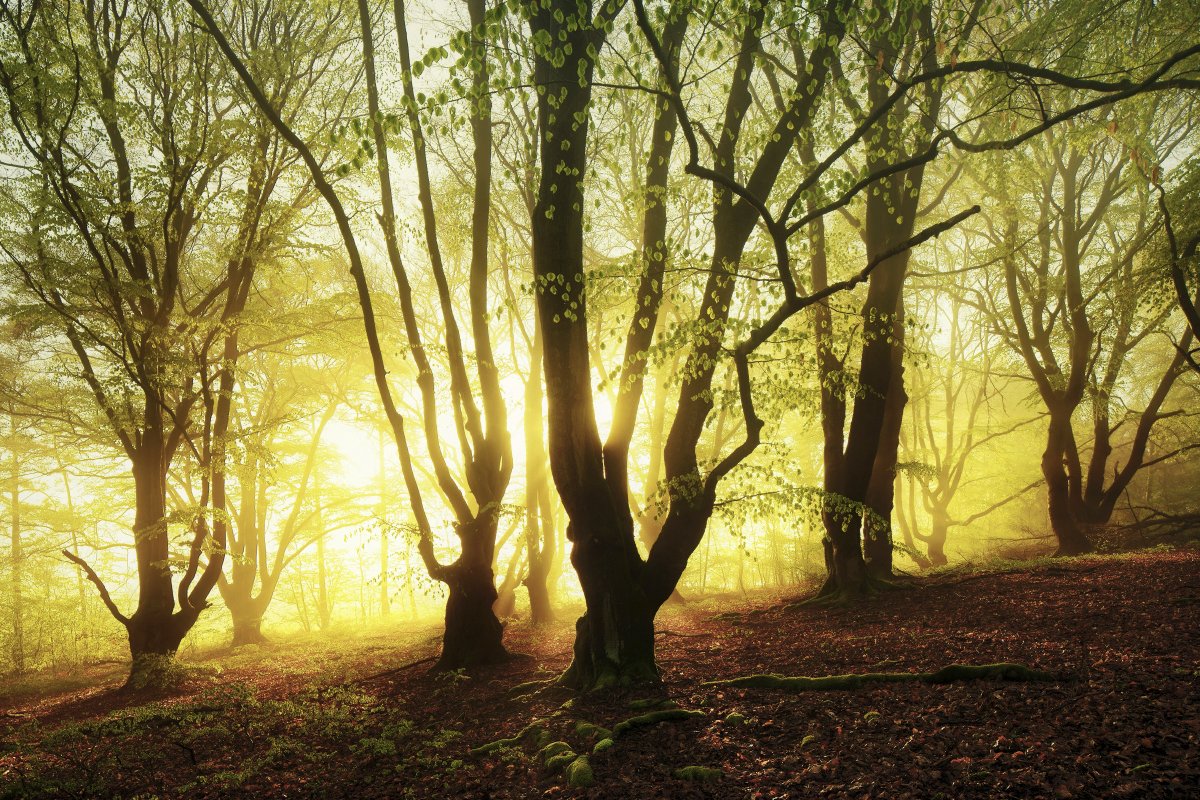This atmospheric and relaxing photograph captures a whimsical forest scene, likely during either sunrise or sunset. The image features about ten trees both in the foreground and background, with sparse yet greenish foliage predominantly at the tops. The sunlight peeks through the dark, shadowy limbs of the trees, casting a serene yellow glow against a grayish-blue sky. The ground, covered in reddish-brown hues likely from fallen leaves and exposed tree roots, adds to the enchanting woodland atmosphere. The scene is both spacious and outdoorsy, evoking a sense of tranquility and natural beauty.